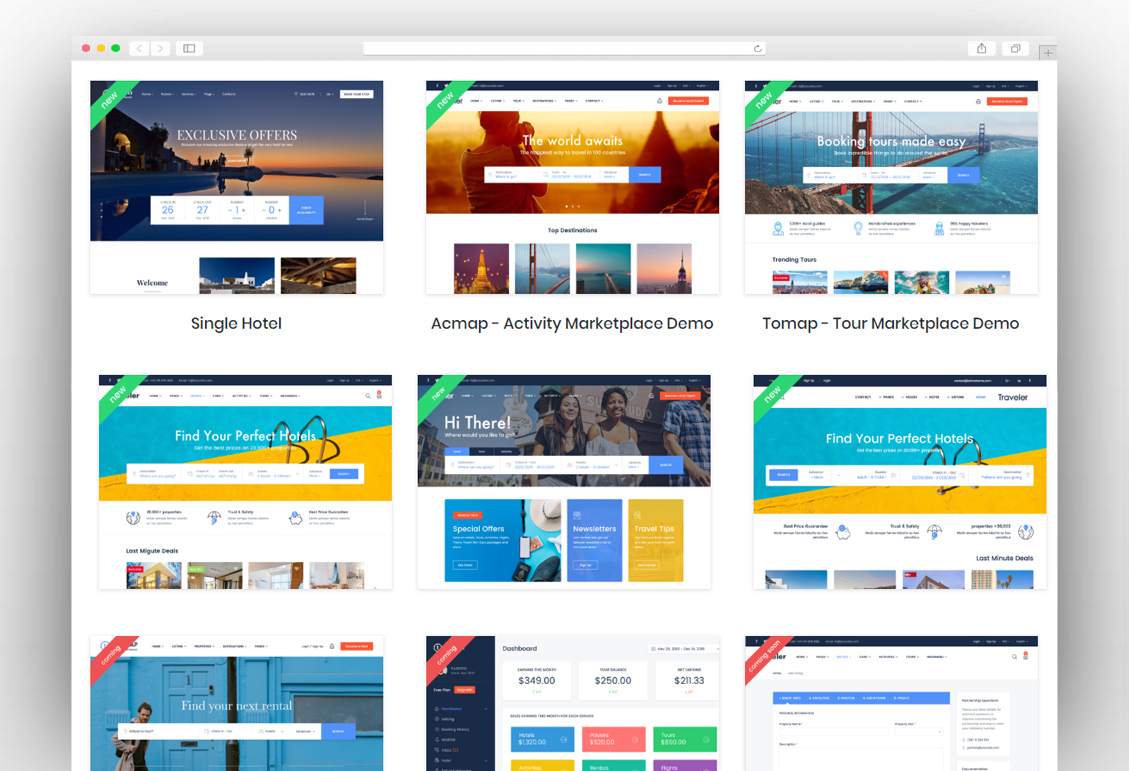The image depicts a section of a website designed to help users create their own customizable website templates. At the top of the screen, there is a search bar accompanied by red, yellow, and green buttons, along with forward and backward navigation arrows. The interface showcases several new website templates, each providing specialized features. 

Highlighted among them is a "Single Hotel" template, prominently marked with a "New" banner and advertising exclusive offers. Additionally, there are templates for an "AC Map," a "Comap Activity Marketplace Demo," and a "Tomap Tour Marketplace Demo," all indicated as new releases. Another key template, "Find Your Perfect Hotel," is also marked as new multiple times in the list.

Further down, there are mentions of additional upcoming templates labeled as "Coming Soon." The primary function of this webpage appears to be offering users a variety of website templates to choose from, each tailored for specific purposes. Once a user selects a template that fits their needs, they can start building their own website based on the chosen design.